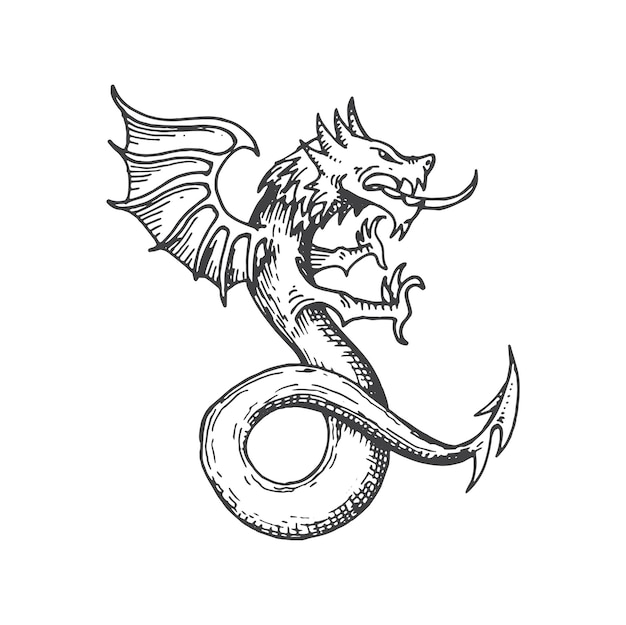This black and white hand-drawn image depicts a detailed dragon, suitable for tattoo art. The dragon's slender, serpentine body resembles that of a snake, adorned with scales. It features two large, sharply clawed arms, akin to bird's talons, and possesses a single visible wing with sharp points on the edges, curling upwards with an inward sharp point. The dragon's head, situated at the top of the image, is equipped with four sharp horns, an open mouth showing rows of jagged teeth, and a long, curled tongue. Its tail, resembling the blade of a curved knife, spirals towards the bottom right, culminating in a pointed tip. The background of the image is left plain white, emphasizing the dark gray, black marker outlines of the dragon.